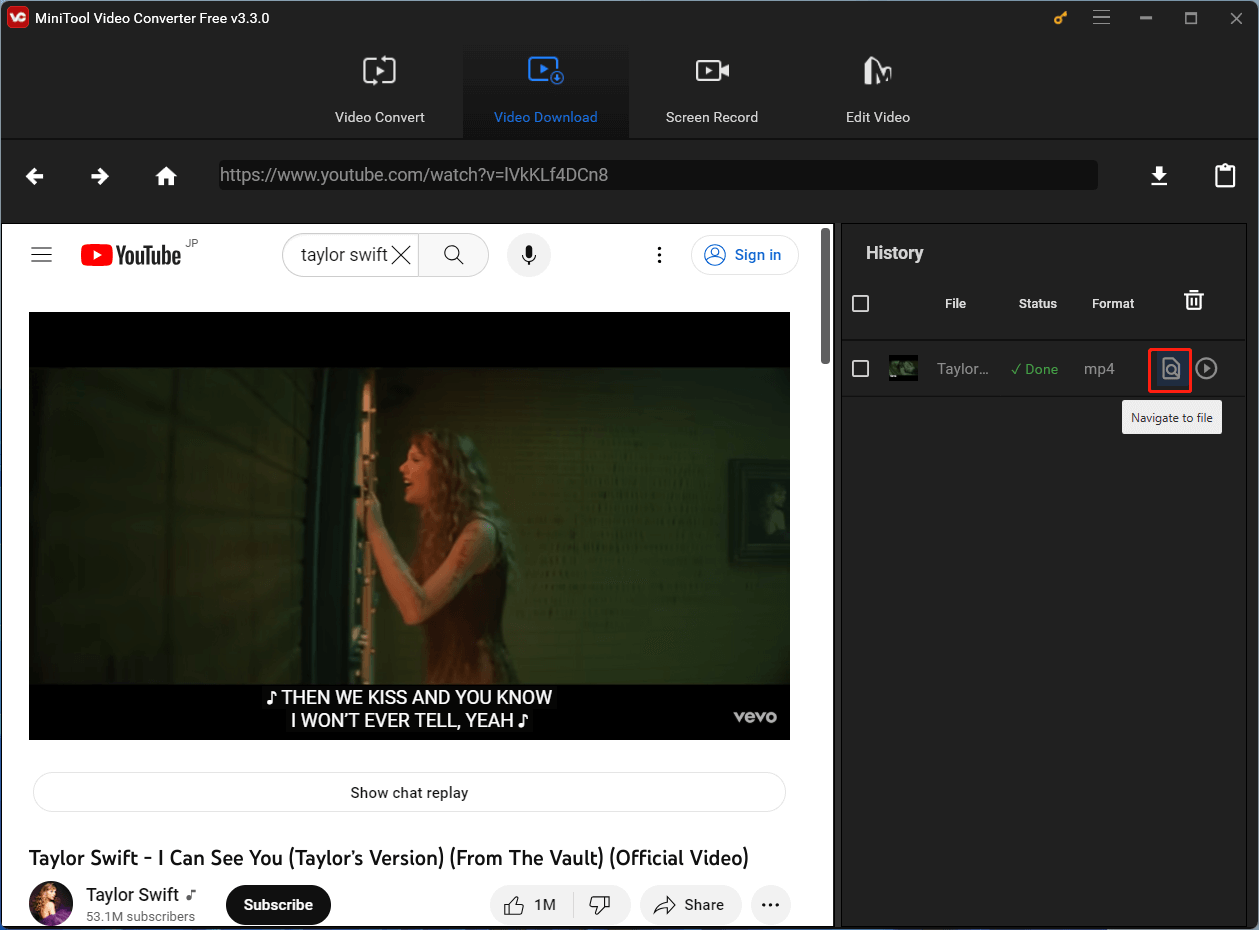A detailed image caption describing the user interface of MiniTool Video Converter Free, version 3.3.0:

---

The interface of MiniTool Video Converter Free, version 3.3.0, is shown. At the top left corner, the application name and version are displayed. Below this, central to the screen, there are several options: "Video Convert," "Video Download," "Screen Recorder," and "Edit Video," with "Video Download" highlighted in blue. Further below and to the left, there are navigation icons: a left-pointing arrow, a right-pointing arrow, and a house icon. 

A search bar with an initial "HTTPS" is located centrally, featuring a "Download" button and a clipboard icon on its right side. To the right of this search bar, there is a YouTube section displaying a thumbnail of Taylor Swift with a sign-in icon next to it. 

Below this, a still image from a Taylor Swift video is visible, captioned with the lyrics, "Then we kiss, and you know I won't ever tell. Yay." A musical note symbol precedes the lyrics. To the right of the image is the Vevo logo. Below, there is an option to "Show Chat Reply," followed by another Taylor Swift video titled "I Can See You (Taylor's Version) (From the Vault) [Official Video]." 

Additionally, the screen reveals that Taylor Swift's YouTube channel has 53.1 million subscribers, accompanied by a "Subscribe" button. Outside the main content area, on the far right, there are options labeled "History," "File," "Status," and "Format."

---

This captures the interface's various visual elements and their respective positions and functions, providing a clear and comprehensive description.